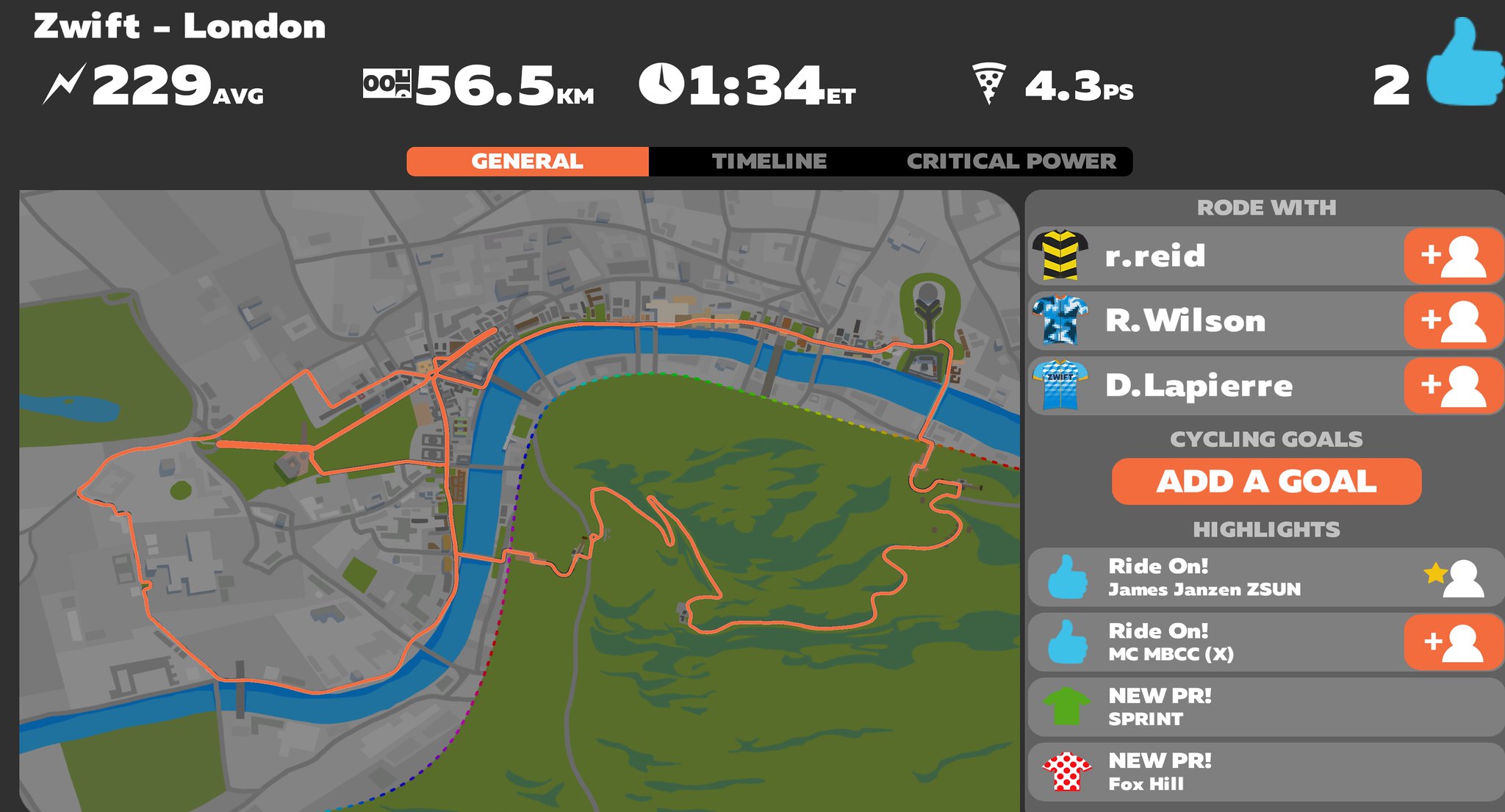The image depicts a computer screen displaying a virtual cycling session on a platform called "Zwift" in London. In the upper left corner, the screen indicates an average speed of 56.5 kilometers per hour, with a duration of 34 minutes and a power output of 4.3 PS, symbolized by a lightning bolt icon. A blue thumbs-up icon with the number two is also visible, indicating positive feedback. The main area of the screen shows a detailed, colored map featuring streets, a river, and grassland, with the user's route highlighted in orange. Additionally, it lists other cyclists who participated in the session: R. Reed, R. Wilson, and D. Lapierre. Below the map, there's a section titled "Cycling Goals" with options to add new goals, along with mentions of achieving a new personal record for sprints and on Fox Hill.